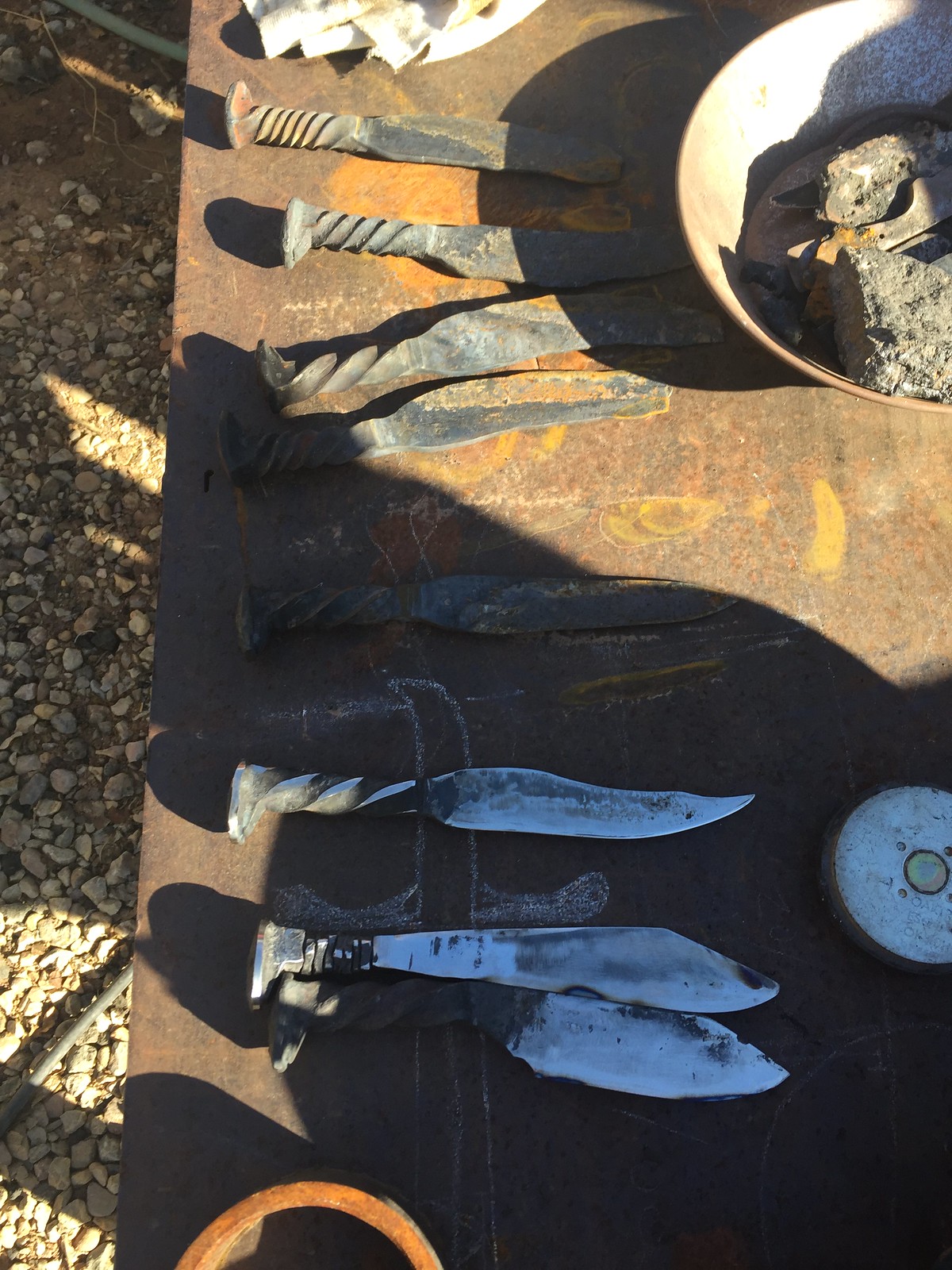The photo appears to be taken outdoors, showcasing a rustic and weathered scene. In the foreground, there is an old, rusty table with areas of rust showing as orange patches. Scattered across the rocky and dirt-laden ground beneath the table, shadows cast by the sun indicate the presence of people nearby. On the table's top right corner sits a bowl containing several large, dark gray rocks with noticeable indentations. Additionally, about eight iron knives are spread across the table; these knives are approximately four inches in length with sharp, silver blades and twisted iron handles designed for better grip. The table also contains what seems to be unfinished knives or old screws with twisted tops. The sunlight streaming through casts an intricate play of shadows over the entire setup, adding depth to the textured scene.